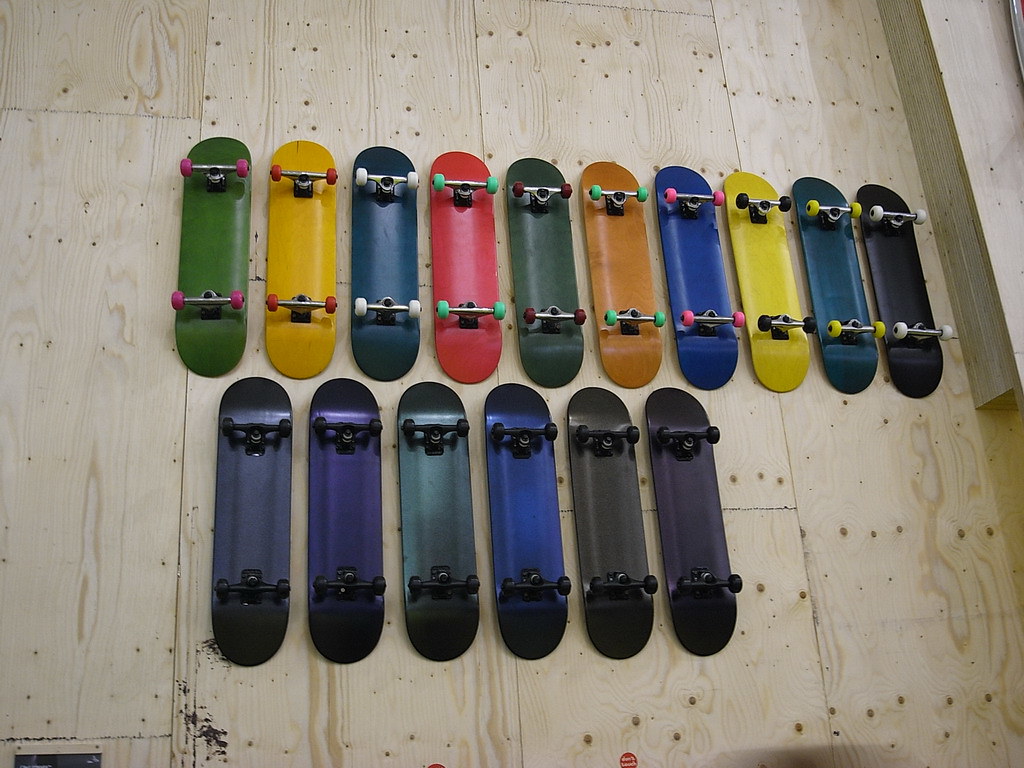This image features a collection of sixteen skateboards laid out in two distinct rows on a light brown plywood floor. The plywood exhibits visible grain patterns and is nailed together, covering the entire background of the photo. The skateboards are positioned upside down, displaying a vibrant array of colored decks and wheels.

The top row showcases ten skateboards with the following deck colors, from left to right: green, yellow, various shades of blue (including turquoise and royal blue), red, dark green, brown, another blue, bright yellow, grayish blue, and black. The wheels on the top row vary in color, including red, white, turquoise, black, green, pink (bubblegum), black, yellow, and white.

The bottom row consists of six skateboards in cooler, more neutral colors, from left to right: black, various shades of purple (including metallic and maroonish), deep teal, royal blue, gray, and a dark blue. All skateboards in this row feature black wheels, creating a contrast with the colorful wheels of the top row.

The overall composition and color diversity of the skateboards against the textured wooden floor create a visually engaging and dynamic image.